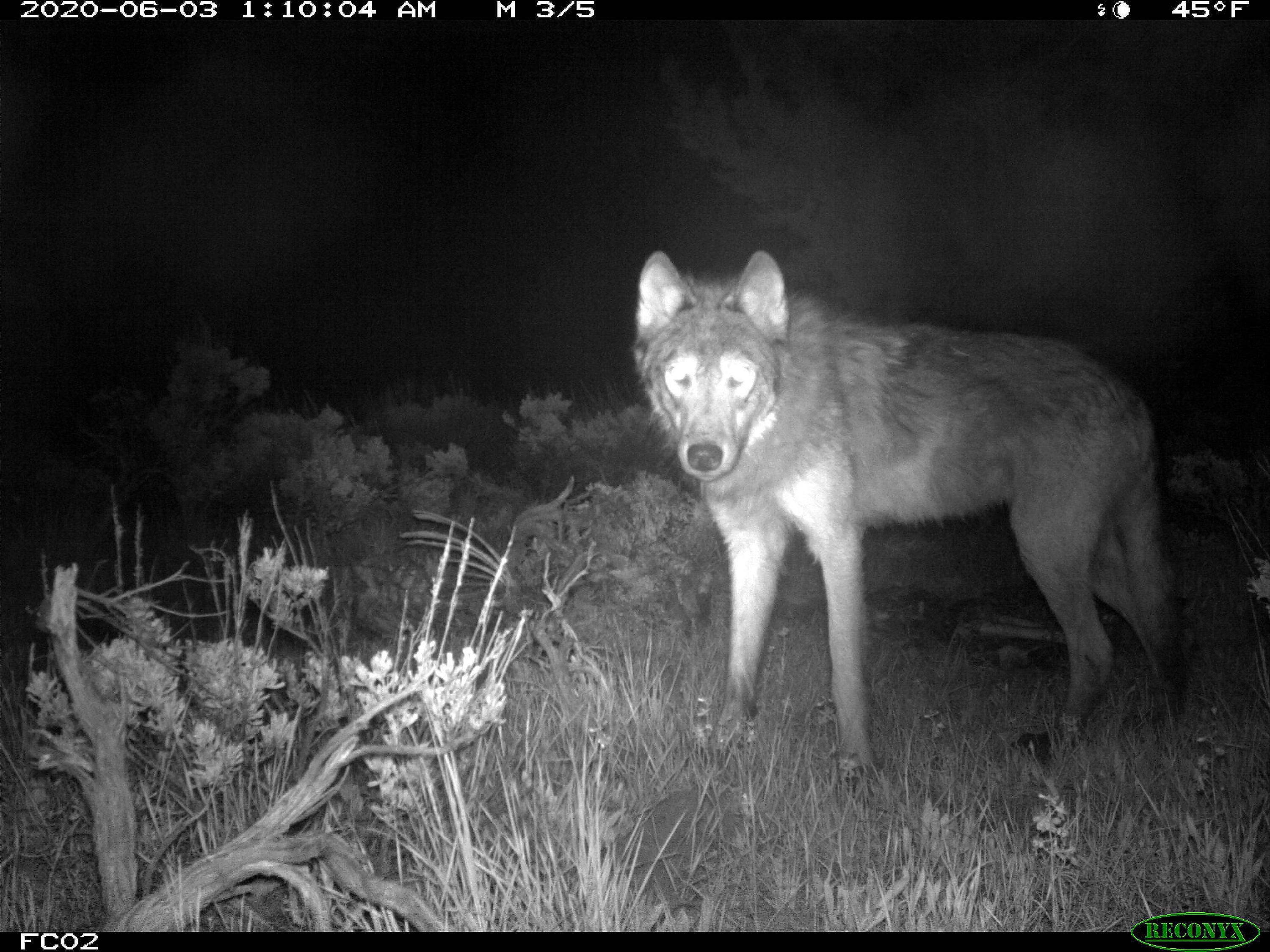Captured by a Reconyx trail camera on June 3, 2020, at 1:10 a.m. with a temperature of 45 degrees, this black-and-white nighttime image features a wolf illuminated by the camera's flash in a sparsely vegetated area. The wolf stands motionless in medium-length grass, surrounded by a few small scrubby bushes and sparse vegetation, including a small flowering bush on the left side. The background is dark, suggesting a remote outdoor location, potentially within a wooded area or brush. The bottom left corner of the image displays "FCO2," while the bottom right corner features a watermark "RECONYX" written in green within a circle. The flash highlights parts of the wolf and its immediate surroundings, possibly triggered by the animal crossing a motion sensor.